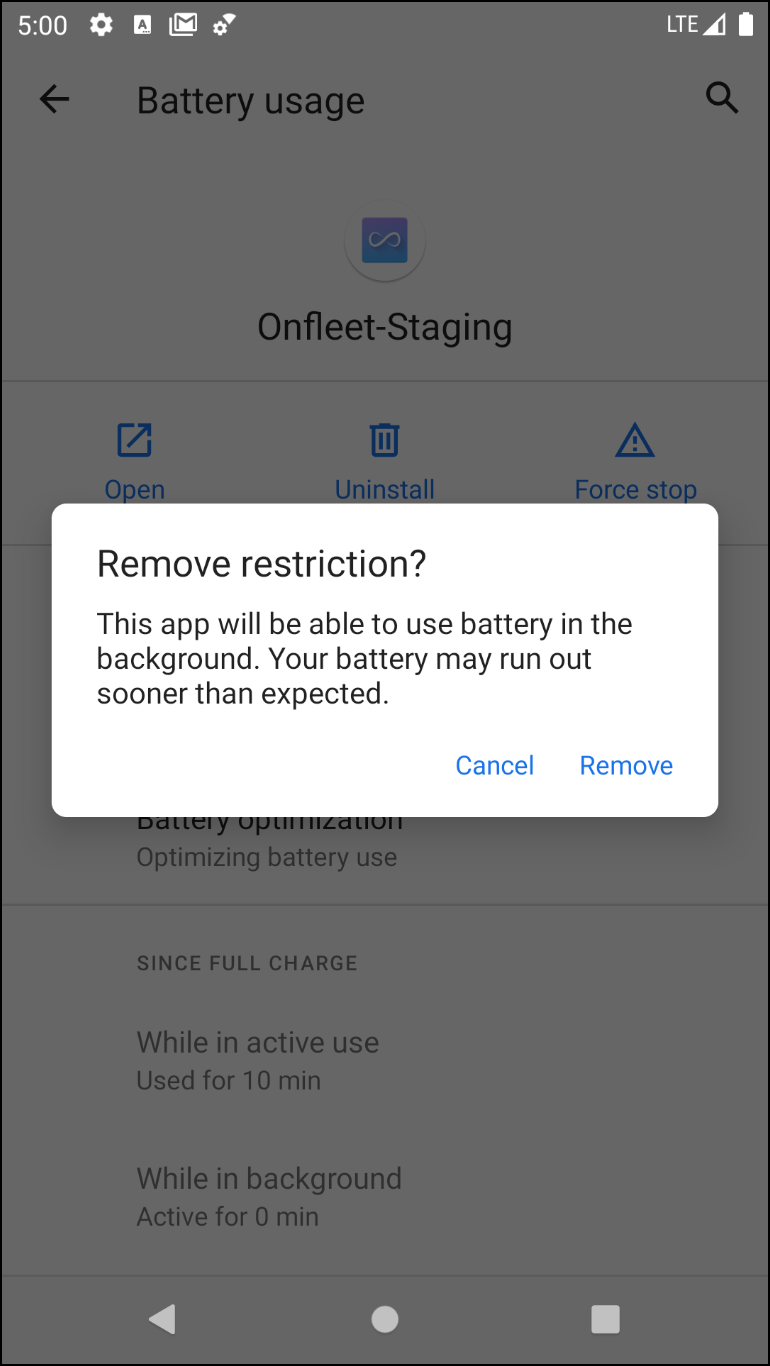The image captures a smartphone screen displaying the “Battery usage” section within the device settings. The settings header is prominently featured at the top, indicating the current time of 5:00 PM. The screen shows that the device is connected to Wi-Fi and has a fully charged battery.

The focus of the image is on an application named "On Fleet Staging," which appears to be configured to manage battery usage. A semi-transparent white dialog box overlays the app settings, presenting a prompt that reads: "Remove Restriction? This app will be able to use battery in the background. Your battery may run out sooner than expected." This dialog offers two options, likely to either confirm or cancel the removal of the restriction.

Below the dialog, additional details about the app's battery usage are partially visible. It indicates that the app has been active for 10 minutes while in use, but it has not consumed any battery while running in the background.

The navigation bar at the bottom of the screen features three icons: a circle to return to the home screen, a left arrow for navigating back to the previous screen, and a square whose function is not determined from the given description.